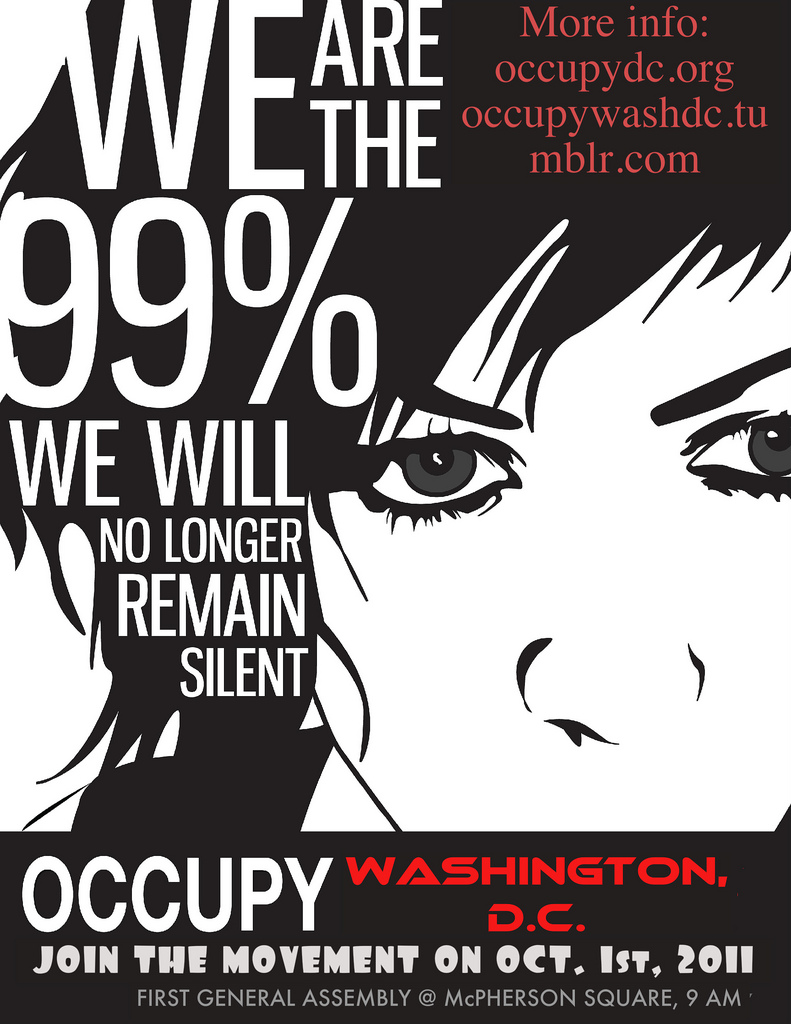This image is a highly stylized protest flyer for Occupy Washington DC. The main focus of the black-and-white illustration is a close-up of a woman's face with jaggedly cut short hair and dark gray irises. Her black hair forms the backdrop for white text on the left side, which reads: "We are the 99%. We will no longer remain silent." In the top right corner, red text within her hair provides further information, stating: "More info: OccupyDC.org, OccupyWashDC.tumblr.com." At the bottom of the poster, a black horizontal banner features "Occupy" in white text and "Washington DC" in red. Beneath this, additional white text reads: "Join the movement on October 1st, 2011. First General Assembly at McPherson Square, 9 a.m."